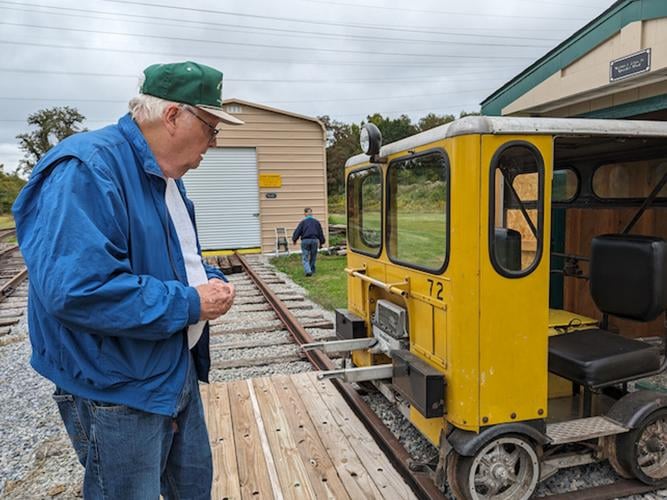In the photo, an elderly man, likely in his late 60s or early 70s, is intently examining a small piece of equipment parked beside some train tracks. He is dressed in a blue jacket, a white sweatshirt, and blue Levi's denim jeans, and he sports a green and yellow baseball hat. His attire is complemented by glasses and white hair. The equipment he is observing appears to be a trolley with a goldish yellow front, featuring two square windshields, a round headlight with a clear lens in a black casing, and a white roof. This trolley, resembling a forklift, has one simple seat with a seat cushion and a small back cushion, and it moves on steel wheels. The equipment is likely used for transporting items along the railroad. In the background, another elderly man is walking toward a garage, possibly preparing to open it for the first man to utilize the trolley for transporting goods or perhaps for maintenance work on the railroad.